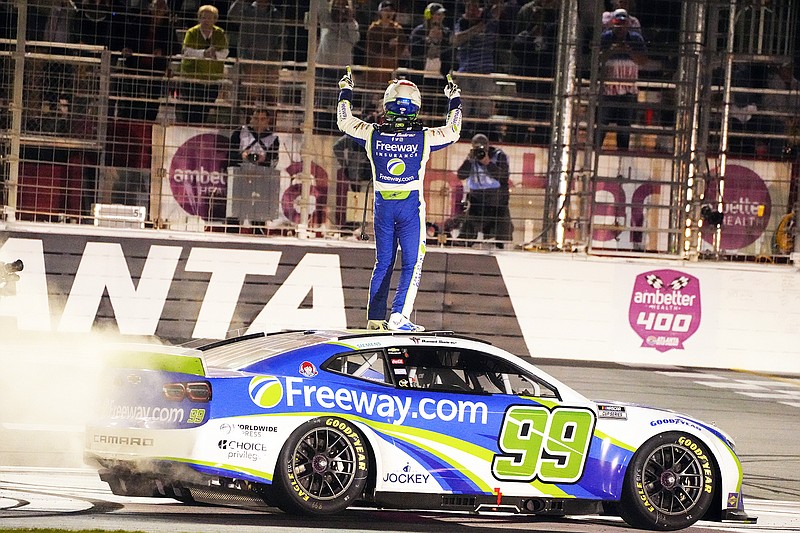In this dynamic photograph, a race car driver stands triumphantly on the roof of their NASCAR-style vehicle, positioned on a racetrack. The car, adorned with Goodyear tires, sports a white, blue, and yellow body featuring a striking red curved stripe that runs diagonally across it. The prominent number "99" appears in green text, outlined in black, on the front door. Sponsorship details include "Freeway.com" in bold white letters across the car's side. The driver, facing away from the camera, wears a blue and white racing uniform emblazoned with "Freeway Insurance" on the back, along with a white helmet.

The celebratory mood is evident as the driver points both index fingers skyward, signaling victory, while looking towards the packed stands behind a fenced area. The background includes the signage "ANTA" and "Ambetter 400" within a pink shield, indicating the event. Smoke rises from the car's rear, adding to the high-energy atmosphere of the photograph.